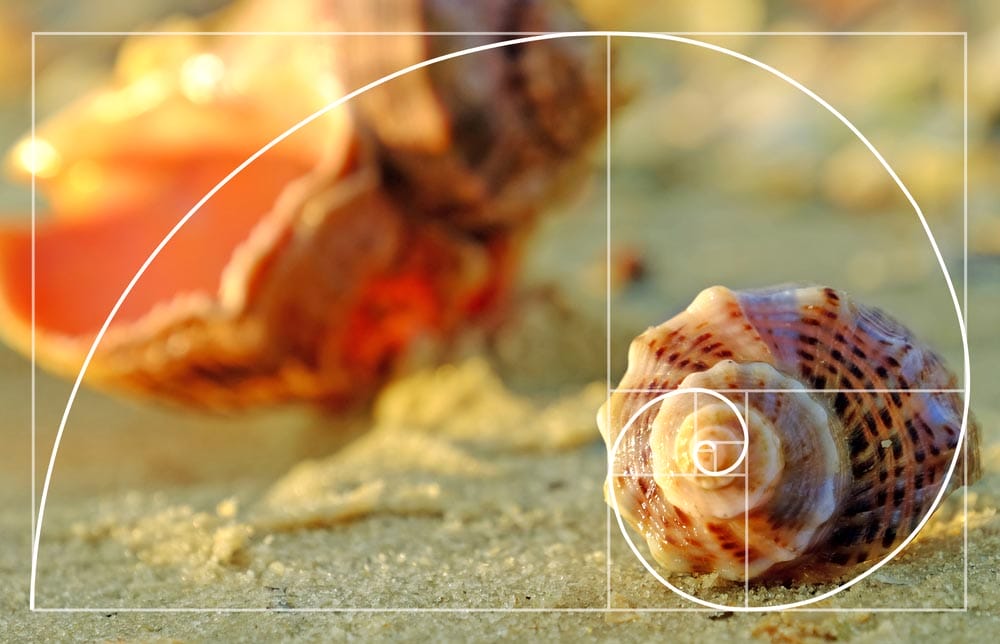This photograph captures a serene beach scene featuring two conch shells resting on the sand. The foreground displays a small, detailed conch shell positioned towards the bottom left corner, with its spiral intricately facing the viewer. In contrast, the background showcases a larger, upside-down conch shell near the top left, slightly blurred to emphasize depth. Superimposed on the image is an elegant white spiral design, reminiscent of a rolling wave, that gracefully loops across the entire scene, echoing the natural spiral pattern of the shells. A thin white rectangular border frames the entire composition, introducing a structured yet harmonious element that complements the fluid spiral. This intricate overlay gives the image a polished, almost logo-like appearance, making it well-suited for use in promotional materials or as a sophisticated decorative piece.